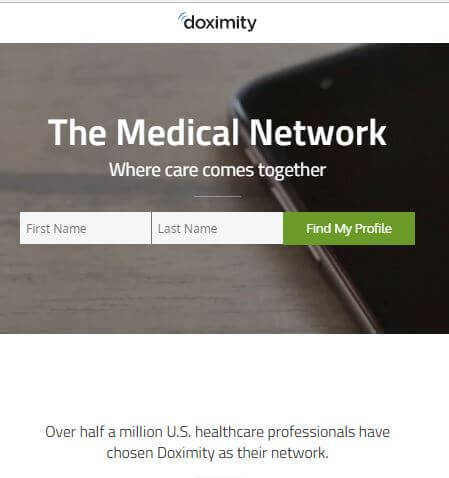In this image from my website "Proximity: The Medical Network Where Care Comes Together," the primary focus is a sleek, modern interface inviting users to engage. At the top of the display, a title banner includes the website's name. Directly beneath this are input fields prompting visitors to enter their first and last names, accompanied by a prominent, green "Find My Profile" button.

Central to the image is a photograph featuring a smartphone, which is switched off with a dark screen, resting on a desk surfaced in medium wood tones. This evokes a professional, organized atmosphere. Just below the phone, white bold text states, "Over half a million U.S. healthcare professionals have chosen Proximity as their network," emphasizing the platform's widespread adoption and trust. This line is underscored by a subtle, yet distinct, white line, adding a graphical element that enhances the design cohesiveness.